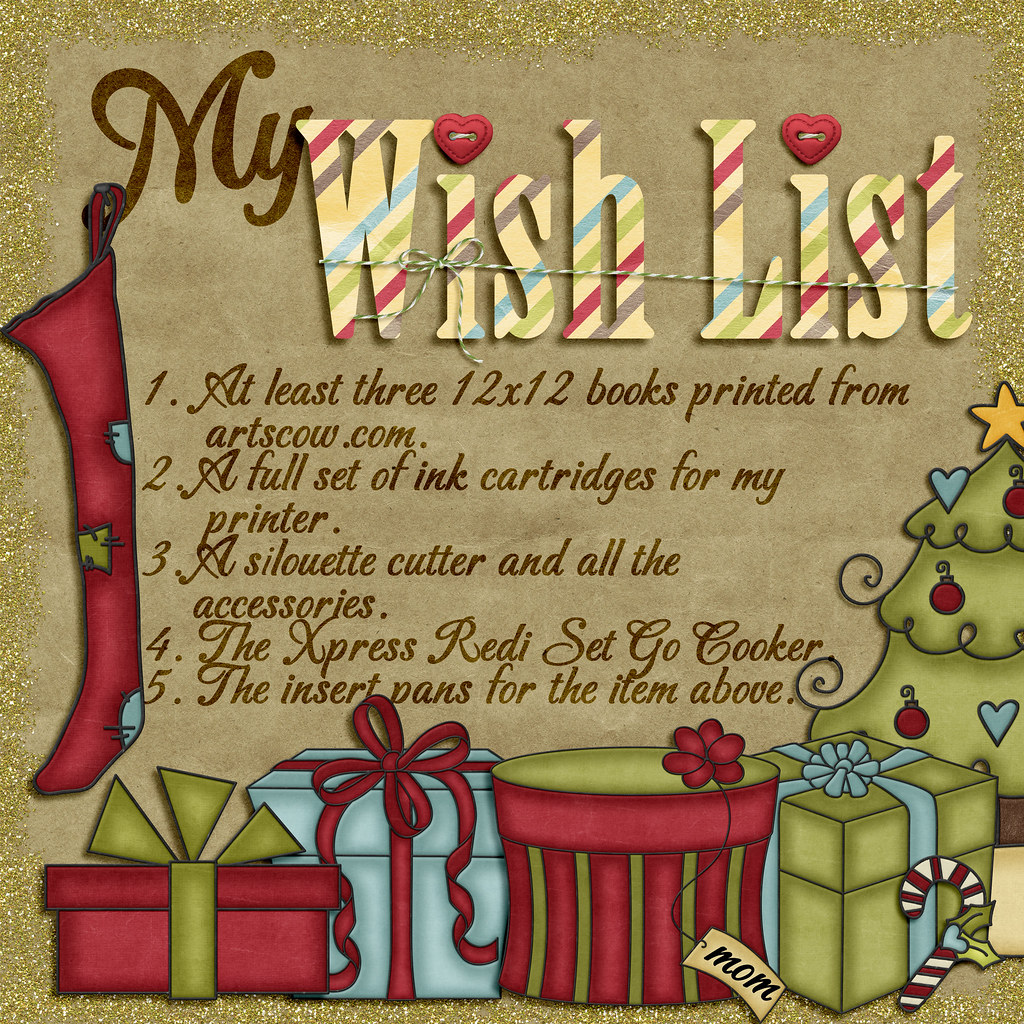This square graphic is bordered by a gold glitter-like frame, with a main background resembling brown paper. At the top, in large dark brown handwritten letters, it reads "MY," followed by "A WISH LIST" in large, multicolored striped letters with diagonal lines. The 'i's in "WISHLIST" are dotted with red heart shapes. This title also includes a three-dimensional effect with a drop shadow and is adorned with a piece of twine tied in a bow. Hanging from the corner of the 'M' is a small stocking. 

Below the title, five handcrafted, dark brown handwritten items are listed:
1. At least three 12x12 books printed from artscow.com.
2. A full set of ink cartridges for my printer.
3. A silhouette cutter and all the accessories.
4. The Express Ready Set Go cooker.
5. The insert pans for the item above.

The lower section of the image features simple illustrations, including a row of gift boxes with one tagged "To mom," a small Christmas tree on the right, and a candy cane. These elements add a festive touch to the overall wish list theme.